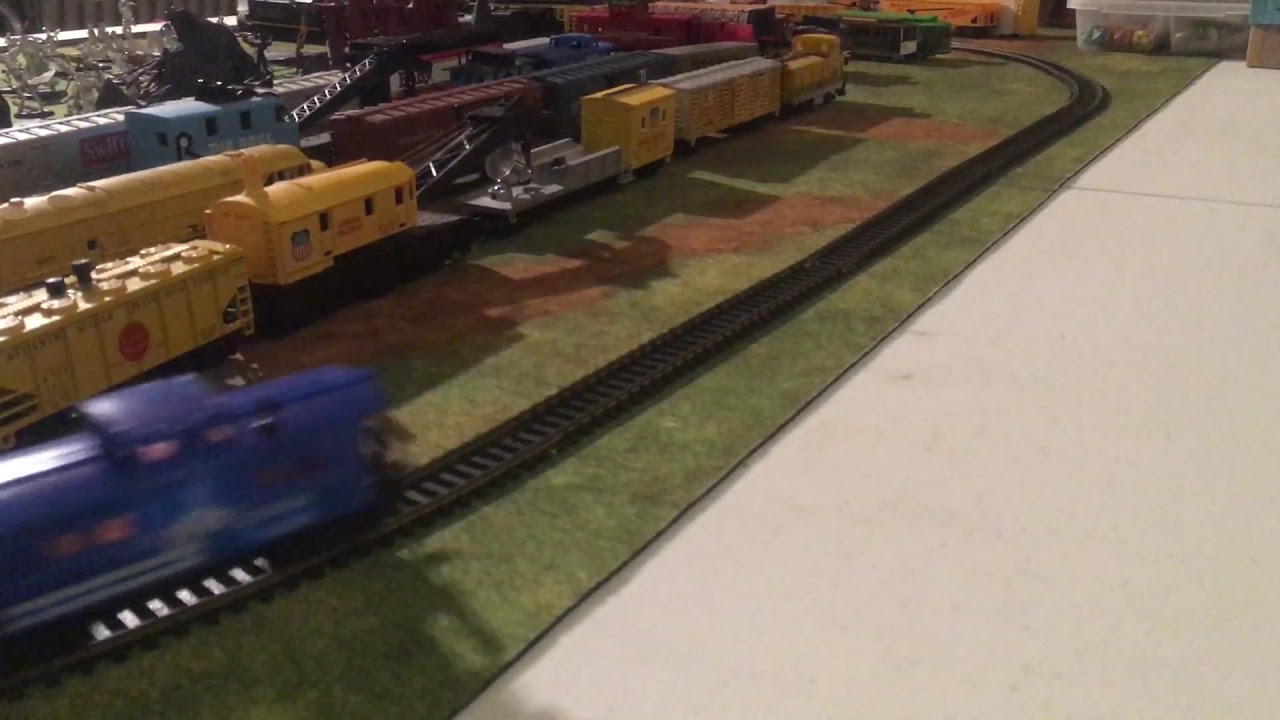This photograph captures an intricate model train layout meticulously set on a green mat positioned on a flat gray surface. Dominating the lower left corner is a blue diesel locomotive, slightly blurred to illustrate its motion along the tracks. Surrounding the active train, numerous other trains and cars populate the scene, highlighting a diverse collection. Immediately to the left of the blue locomotive, a series of freight cars are organized in three sidings. The first siding hosts an ensemble of two yellow boxcars, a flatbed, another two yellow cars, and a caboose. The central siding features a yellow boxcar alongside a brown boxcar, while the third siding displays additional boxcars flanked by what appears to be a miniature house. Throughout the layout, the intricate network of tracks spans the green surface, suggesting a complex and expansive diorama dedicated to model railroading. A patch of visible white flooring on the right further frames this detailed miniature world, emphasizing its scale and the hobbyist's attention to detail. There are no people or text in the image, reinforcing the focus on the trains and their layout.